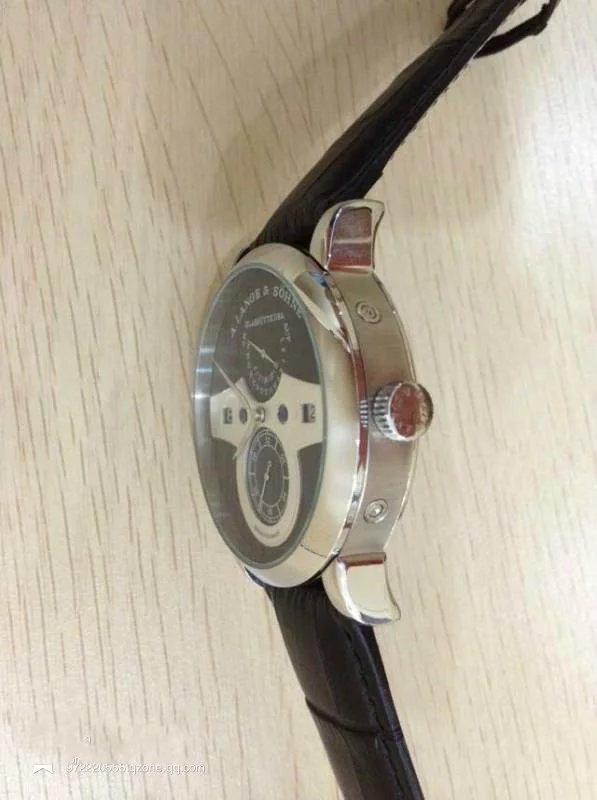The image showcases a detailed, close-up photograph of a watch placed on its side on a nearly white, subtly textured table. The watch features a black band, which appears to be either leather or plastic, with the top strap positioned at the upper part of the image and the bottom strap at the lower part. The watch face, oriented toward the left, is encased in a silver frame and covered with glass, giving it a sleek, polished look. The face itself is black, adorned with two smaller circular sub-dials separated by a rectangular section in the middle, possibly indicating different time zones or additional functionalities like a date display. The crown, used for setting the time, is located at the top right of the watch face. The table surface underneath highlights a light gray color with fine, continuous lines and texture. Overall, the combination of the watch's design elements—a silver bezel, black band, and intricate face details—creates a visually appealing and sophisticated timepiece.